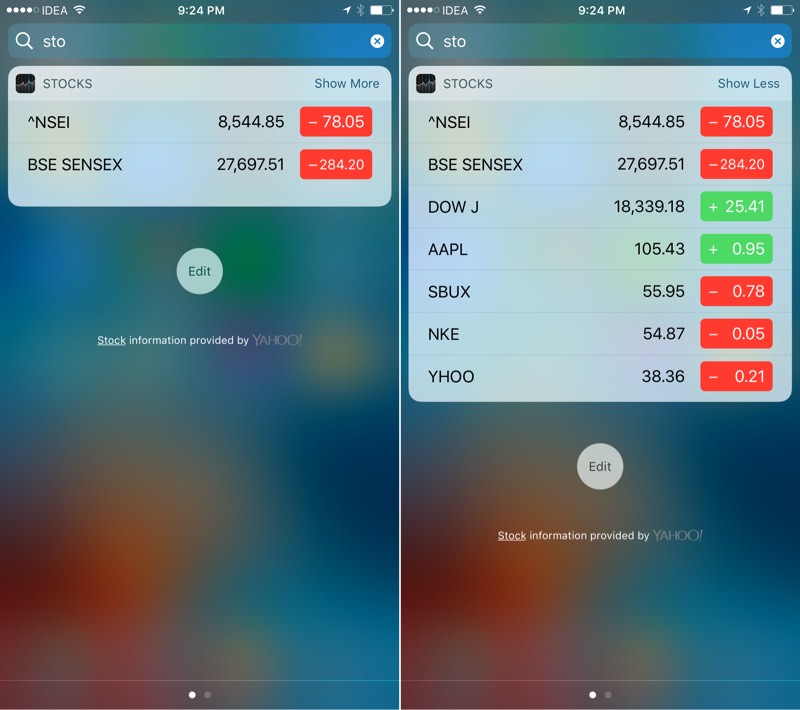The image comprises two mobile phone screenshots displayed side by side, with a background featuring a blurry, translucent blend of colors, predominantly blue, rendering the home screen indistinct through the overlay of pop-up menus.

**Left Screenshot:**
- At the top, a search field displays the text "STO" in white font.
- Directly beneath, a menu entitled "Stocks" appears with a white bar labeled "Stocks" in gray font, and an option for "Show More."
- Following this are two translucent gray entries:
  - The first entry contains:
    - "SEI" marked with a black upward arrow.
    - A value of "8,544.85."
    - A red rectangle displaying "-78.5" in white font.
  - The second entry includes:
    - "BSE SENSEX" in black font.
    - A value of "27,697.51."
    - A red rectangle with the text "-284.20" in white font.

**Right Screenshot:**
- Similar entries are shown as in the left screenshot, but here the section is expanded to display five additional entries beneath the initial ones.

This cleaned-up description aims to provide clarity and detail regarding the content and structure of the two screenshots.